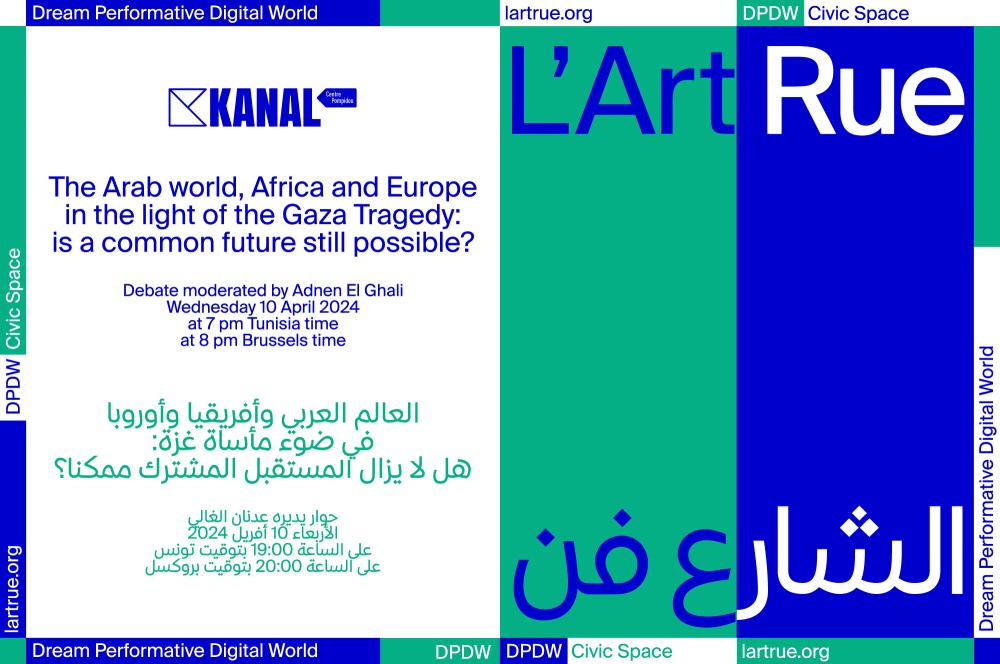The image is a promotional poster divided into three vertical sections: white, green, and blue. The largest section, on the left, features a white background with blue writing that reads "The Arab World, Africa, and Europe in the light of the Gaza tragedy: Is a common future still possible?" Beneath this headline, there is text in Arabic, followed by "Debate moderated by Adnan Al-Khali" and "Wednesday, 10 April 2024 at 7pm Tanzania time, 8pm Brussels time." The middle section has a green background with the text “Dream Performative Digital World” in white, and the name "largetrue.org" in green. The right section is blue and features text in both English and possibly Arabic, including terms like "Civic Space" in blue font and "DPDW" in white font with green and blue backgrounds. The poster combines these elements seamlessly into a single, cohesive horizontal image with promotional and informational content about a scheduled debate.